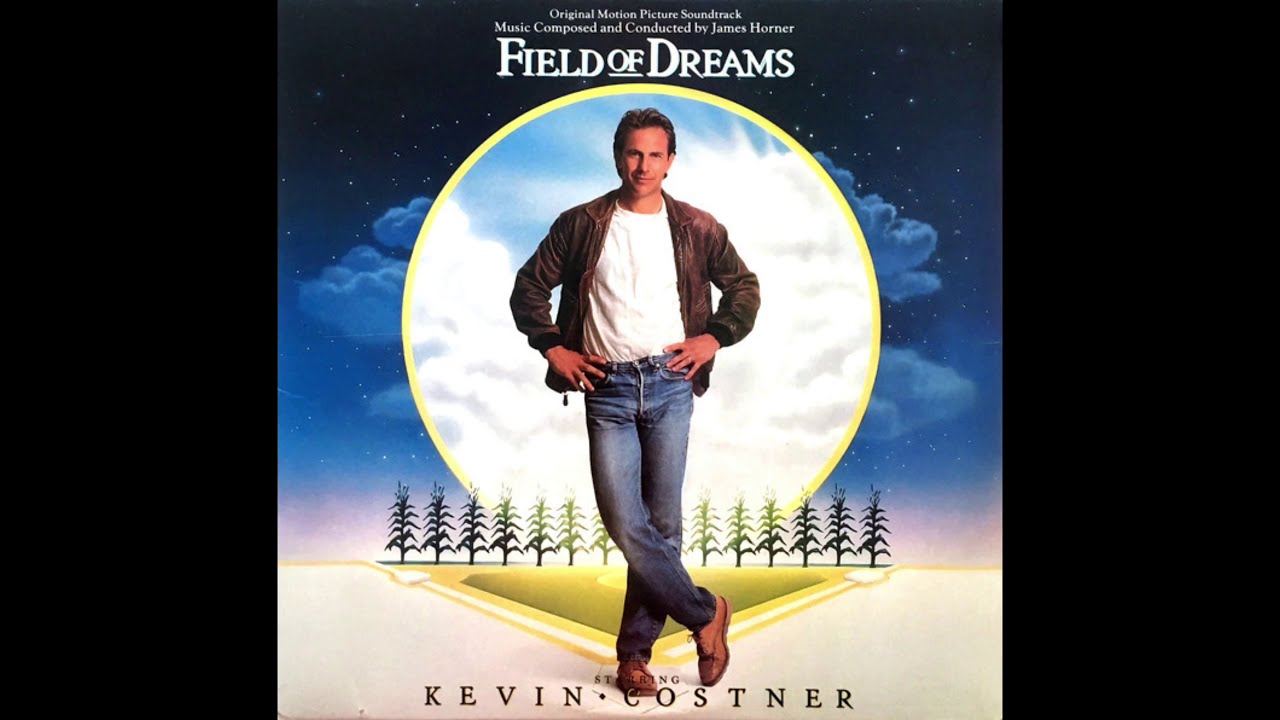This detailed image depicts the cover art of the "Field of Dreams" original motion picture soundtrack. Central to the composition is actor Kevin Costner, standing confidently at the tip of a home plate on a baseball diamond. Costner, clad in a brown leather jacket over a plain white t-shirt, light blue jeans, and brown dress shoes, poses with his hands on his hips, offering a subtle smile. Behind him stretches a row of tall green corn. The night sky forms the backdrop, adorned with a large yellow-outlined moon, scattered stars, and wispy clouds adding a touch of dreamlike ambiance. At the very top of the image, the text reads, "Original Motion Picture Soundtrack, Music Composed and Conducted by James Horner," with "Field of Dreams" in large, bold white letters below it. At the bottom of the image, the caption states, "Starring Kevin Costner" in black font. The color palette is a mix of earthy tones and night-time hues like black, gray, blue, yellow, white, and tan, emphasizing the outdoor, serene setting and giving it a nostalgic and heavenly feel.